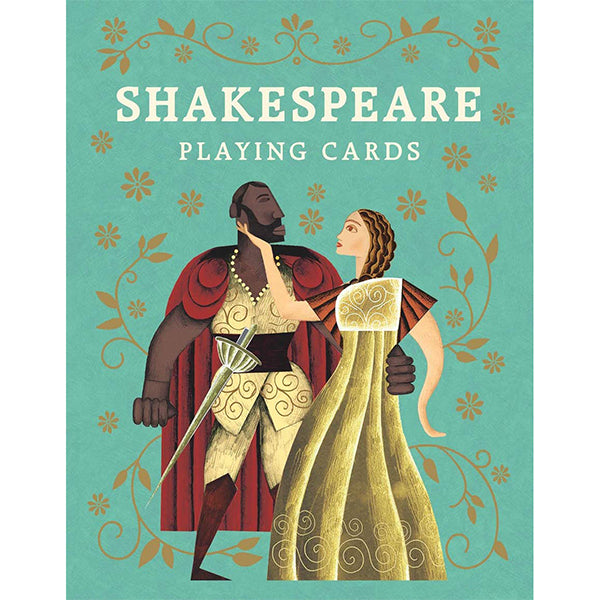The image is a detailed, color illustration of a cover design for a deck of playing cards, prominently featuring Shakespearean characters. Set against a light aqua blue background, the scene is embellished with intricate gold leaf patterns in a restrained Paisley style, featuring twirly, curly cues that resemble leaves and flowers. At the center, two animated, cartoon-like figures are depicted - a black man on the left, dressed in off-white armor with a white sword at his side and a long red cloak draped over his shoulders, and a white woman on the right, wearing a golden gown with an ornate white curvy line design around the bust and orangish-black striped details on the shoulders. She has long, wavy brown hair and red lips, and is holding the man's chin while gazing up at him. The man's arm is wrapped around her waist. The text "Shakespeare Playing Cards" is boldly displayed in white at the top of the image, creating a focal point above the gold flourishes. The illustration combines elements of graphic design and typography to create a visually striking and cohesive cover.